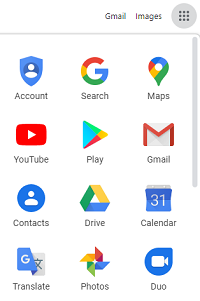The image depicts a grid of app icons against a predominantly white background. At the top, there's a white bar featuring labeled options in black font: "Gmail" and "Images," both with their initial letters capitalized. To the right of these labels, on the upper-right side, there is a gray circle containing nine black dots arranged to form a square, suggesting a menu or app grid icon. Below this top bar, a thin gray horizontal line acts as a separator.

Positioned on the far right side, there's a vertical gray line that appears to function as a scrollbar. The app icons are organized in a neat grid layout consisting of four rows, with each row comprising three app icons. The first row includes icons for "Account," "Search," and "Maps." The second row contains icons for "YouTube," "Play," and "Gmail." The third row features "Contacts," "Drive," and "Calendar." The final row displays icons for "Translate," "Photos," and "Duo."